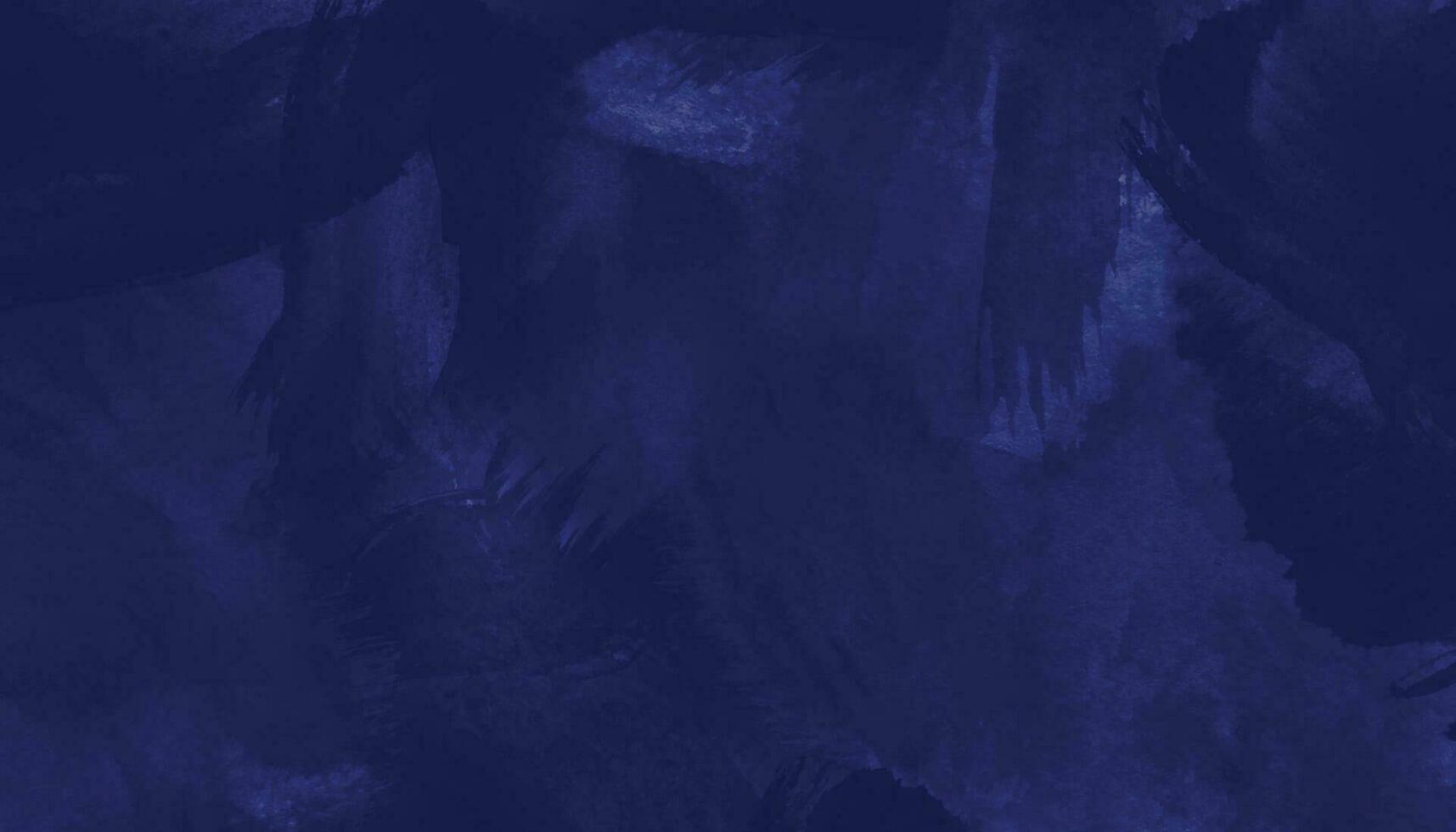This rectangular painting showcases a captivating interplay of various shades of blue, ranging from dark navy to lighter hues, with occasional touches of white. The brush strokes vary in thickness, creating a textured and dynamic surface that gives the piece an abstract quality. Although devoid of any recognizable objects or text, the swirling patterns of paint evoke different interpretations, resembling ocean waves, a starry night sky, or possibly the depths of a forest or cave. The blend of thicker, bolder strokes with thinner, sheer layers enhances the painting's calming and serene atmosphere. This artwork, likely suitable for display in a museum or gallery, invites viewers to find their own meaning within its harmonious swaths of blue.